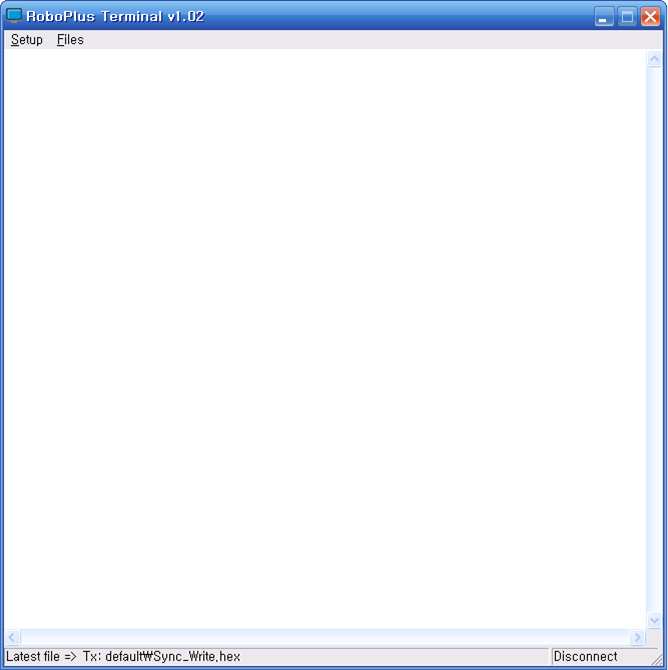This screenshot captures the user interface of the Robo Plus Terminal V1.02 software. The interface features a primarily white background with minimal content. At the very top of the screen, there is a title bar displaying the software name "Robo Plus Terminal V1.02" aligned to the left, with standard window control buttons—Minimize, Maximize, and Close—on the right.

Immediately beneath the title bar, on the right side, there are two navigational tabs: "Setup" and "Files". The central portion of the screen is entirely blank, highlighting its current inactive state.

At the very bottom of the interface, several text elements and controls are visible: 
- A status message that reads: "Latest File = Text; default".
- Next to this, there's a 'W' with a line through it.
- Further right, an option labeled "Sync.Write.Hex" is displayed.
- Finally, there is a "Disconnect" button at the far right of the bottom bar.

This appears to be a troubleshooting or operational terminal within a computer program, yet it reveals no active operations or loaded content in the main viewing area.